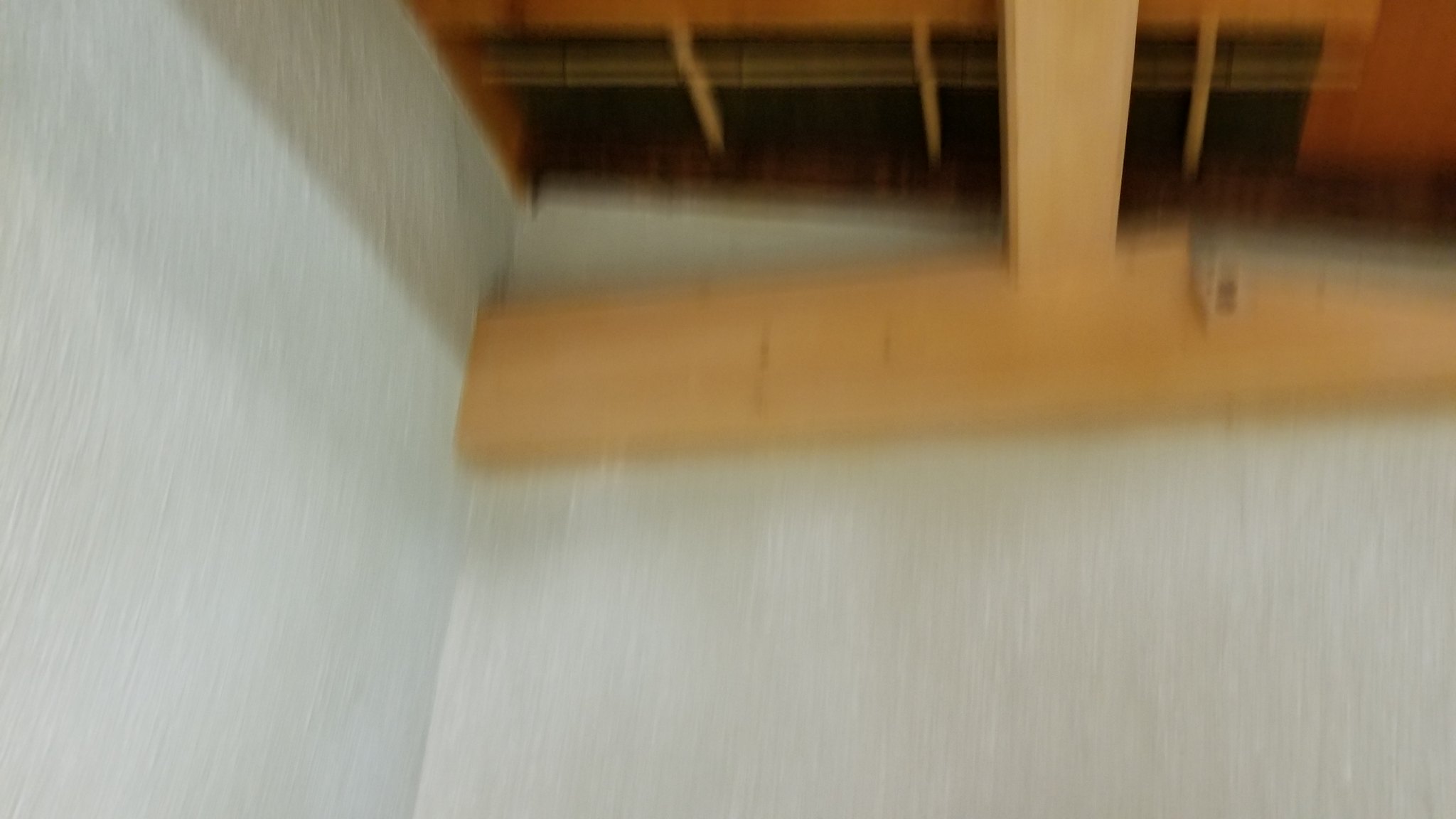This image showcases a very low-quality, blurry color photograph primarily dominated by a white surface. The visible portion of the image captures the intersection where two white walls meet, extending into a corner that transitions to a ceiling. On the ceiling, there appears to be a dark wooden feature, possibly a window frame, composed of rectangular sections. In the foreground, an unfinished wooden structure is discernible, albeit blurred. This structure consists of a vertical wooden plank with another horizontal plank affixed approximately two-thirds up its length. The overall lack of clarity in the photograph makes it challenging to discern finer details.